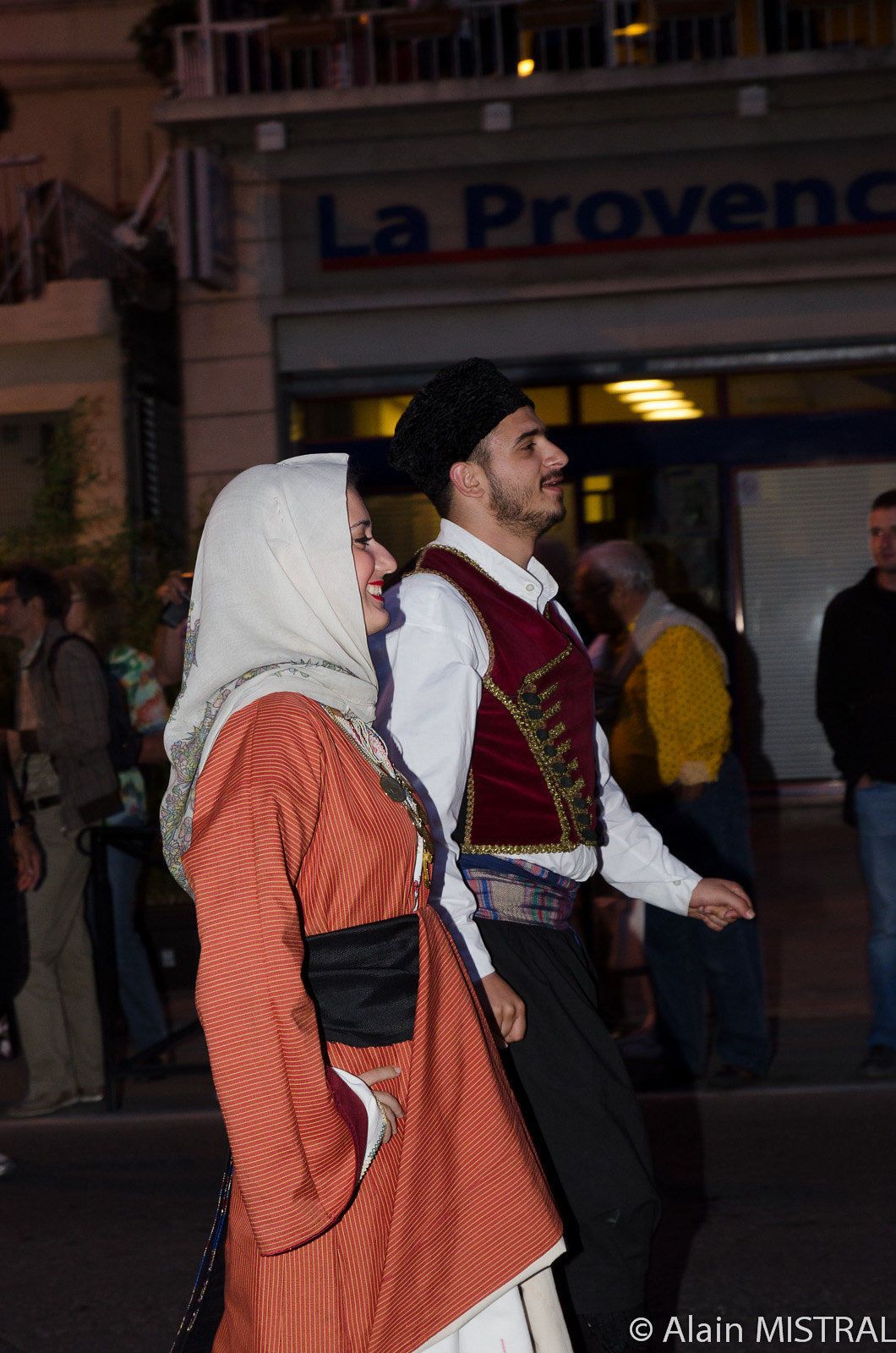A side profile of a woman in a white headscarf that drapes elegantly around her head and down to her chin. She is adorned in an orange jacket or similar garment, accentuated by a black belt around her waist. Her expression is bright and joyful as she gazes forward. Beside her stands a man wearing a black hat, a crisp white shirt, and a rich, velvety burgundy vest embellished with gold trim. He pairs this with black pants. The setting is a nighttime street, with a dark, gray-toned pavement underfoot. In the distance, a sidewalk is visible with a few people standing around. The background features the facade of a building with the sign "La Provence," contributing to the scene with a slightly faded, grayed-out appearance.